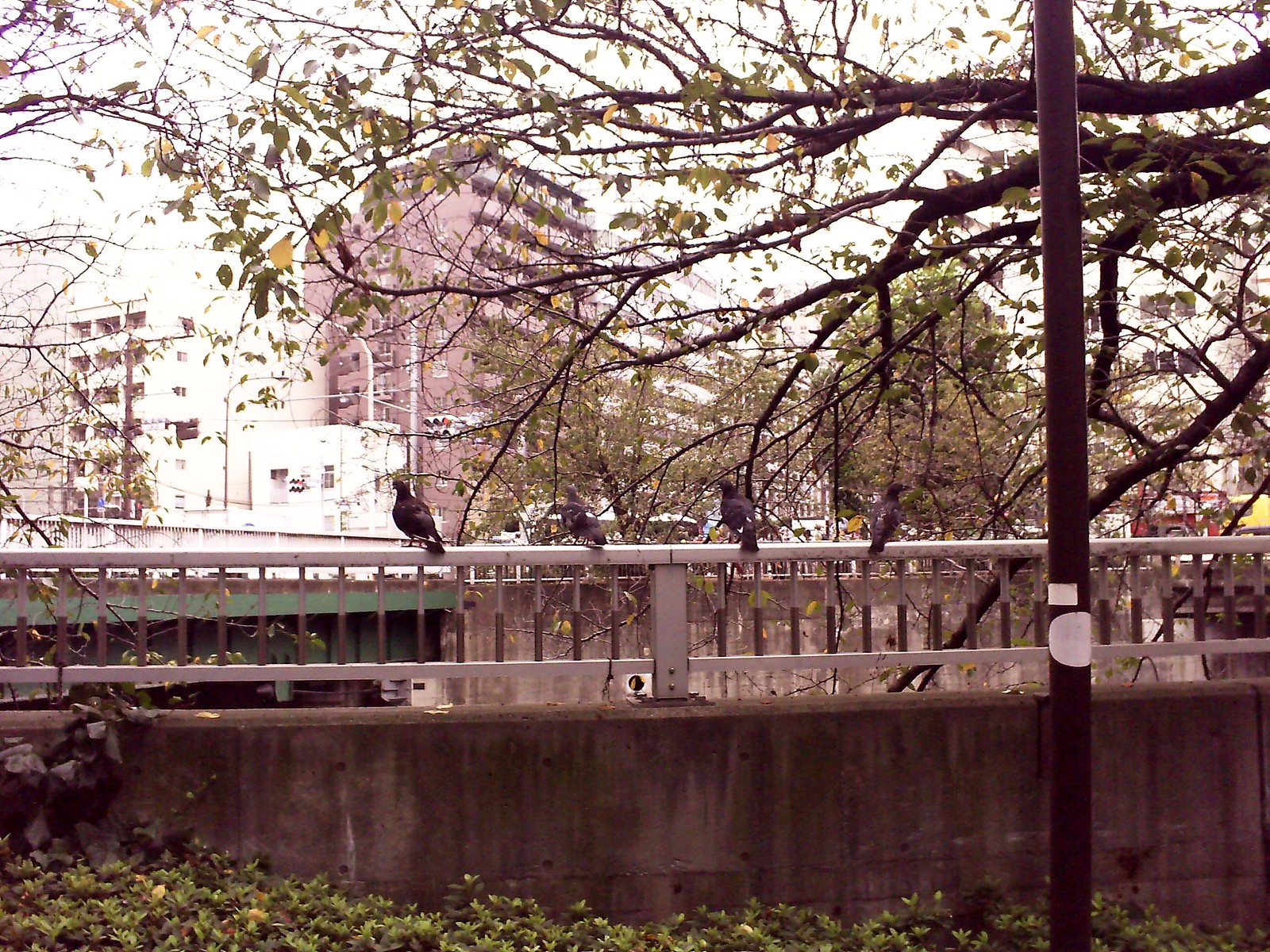This color landscape photograph captures an urban environment on a cloudy day, with a focus on a concrete barrier capped with a metal fence. The barrier is stained and weathered, and the metal fence above is silver in color. Perched almost centrally on the fence are four pigeons, mostly gray and black, all facing away from the viewer. Below the barrier, the ground is strewn with dried, brown and yellow leaves. The background features a mix of high-rise buildings, including a prominent six-story white building and a taller brown structure, partially obscured by a sparsely-leaved tree on the upper left. The tree's branches extend towards the left, their few remaining leaves also brown. A highway or multi-lane road likely lies beyond the barrier, though it remains out of sight due to a dip. Additionally, a utility pole with two white stickers, one square and one circular, stands to the right of the barrier.